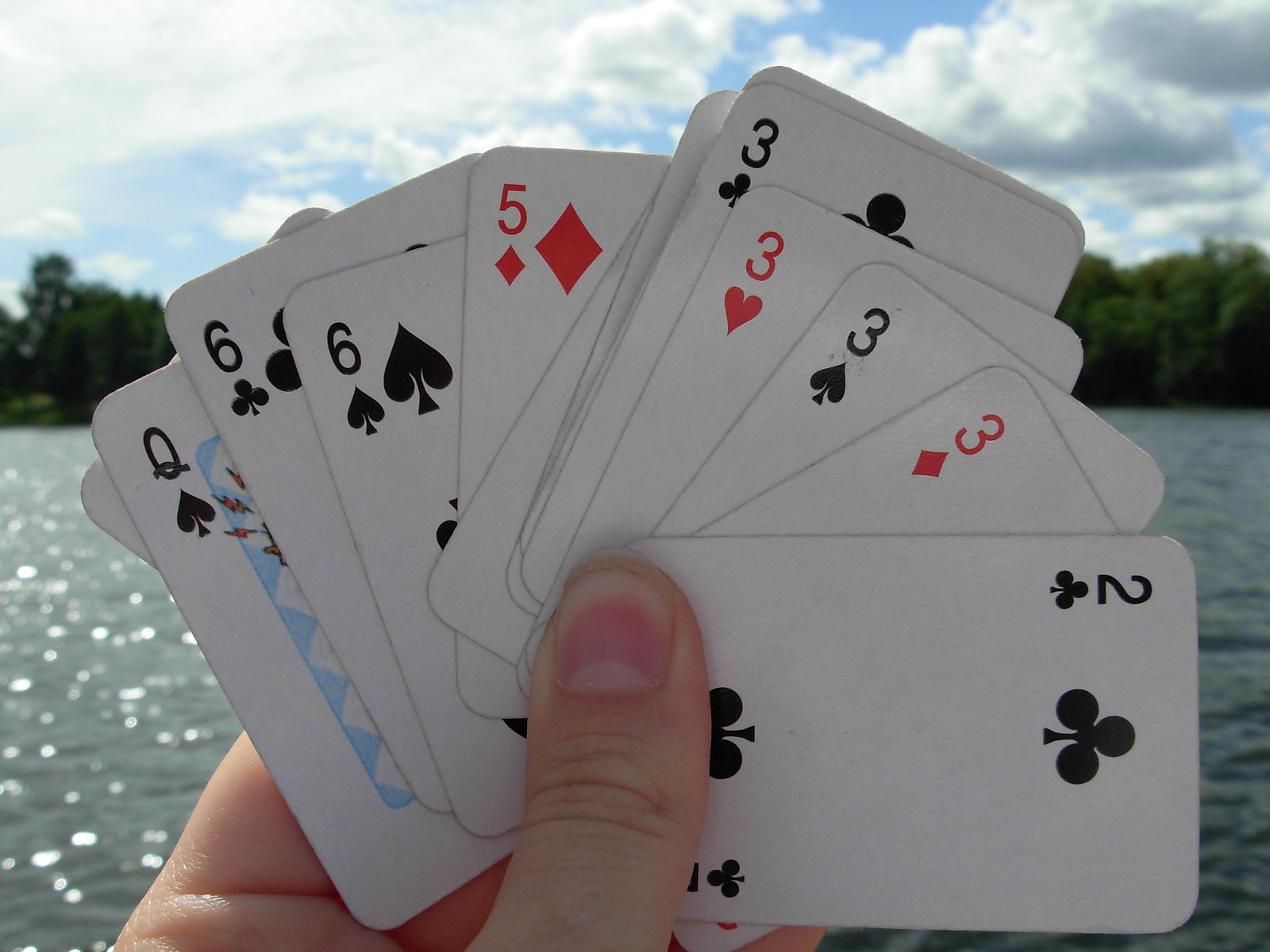A person's left hand is prominently displayed, holding a fan of 13 playing cards while standing in front of a scenic lake. The thumb is visible, anchoring the arrangement of cards. The cards, fanned out in a typical poker grip, show the following sequence from left to right: a hidden card, Queen of Spades, Six of Clubs, Six of Spades, Five of Diamonds, three hidden cards, Three of Clubs, Three of Hearts, Three of Spades, Three of Diamonds, and a Two of Clubs. The individual has lighter skin, and in the background, the tranquil lake with its grayish, brackish water is framed by dark green trees. Above, the sky is a serene blue, dotted with white clouds.